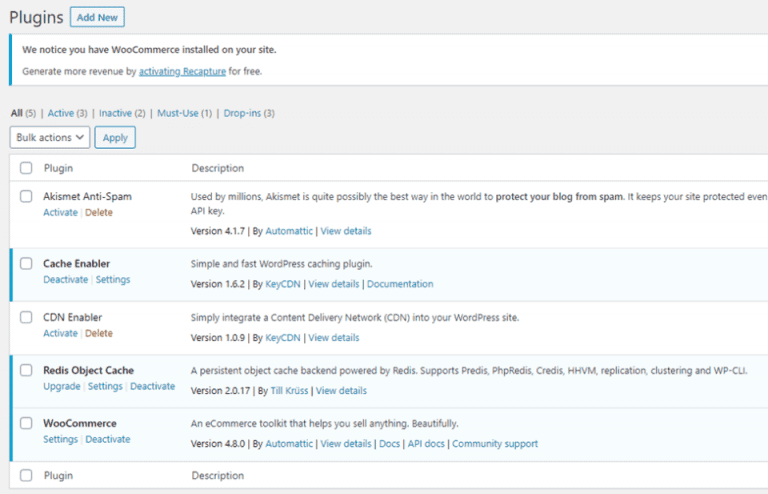The image is a detailed screenshot displaying a webpage or program interface related to plugin management, reminiscent of an Excel spreadsheet with alternating row colors (white, gray, green, and occasionally blue for differentiation). 

In the top left corner, a title prominently reads "Plugins" in black font. Situated next to it is a light green "Add New" button with slightly darker green text. 

Below the title, the first row, shaded in green or gray, highlights an announcement suggesting the installation of WooCommerce to generate more revenue, with a clickable link "activating recapture for free."

Further down, there is another green box containing several filter or menu options: "All", "Active", "Inactive", "Must Use", and "Drop-ins" on the left side. Directly beneath this is a bulk action dropdown menu, accompanied by an "Apply" button.

The interface is organized into columns, starting with "Plugin" followed by "Description", each detailing various plugins. The plugins listed include Akismet Anti-Spam, Cache Enabler, CDN Enabler, Redis Object Cache, and WooCommerce. The descriptions, typically spanning a line or two, are located to the right of each plugin name.